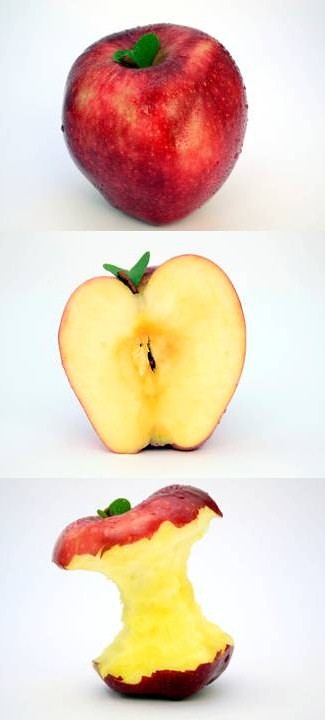This three-part image showcases the stages of a red apple's transformation. In the first picture, taken from a slightly elevated front view, we see a whole, healthy-looking apple, glistening with condensation. The apple is primarily red with hints of yellow and pink, and it's slightly lopsided, giving it a unique charm. A small leaf is attached to the short stem at the top.

The second picture shows the same apple sliced longitudinally in half, exposing its juicy, yellowish flesh and the core with visible seeds. The lopsided nature of the apple is still apparent, and the stem and attached leaf are visible on both halves.

In the third picture, the apple has been eaten completely around, leaving behind a traditional apple core shape. The remnants of the bright yellow flesh surround the core at the top and bottom, contrasting with the darker red skin that remains. The stem and small leaf are still present, attached to the eaten apple core, illustrating the fruit's journey from whole to completely consumed.